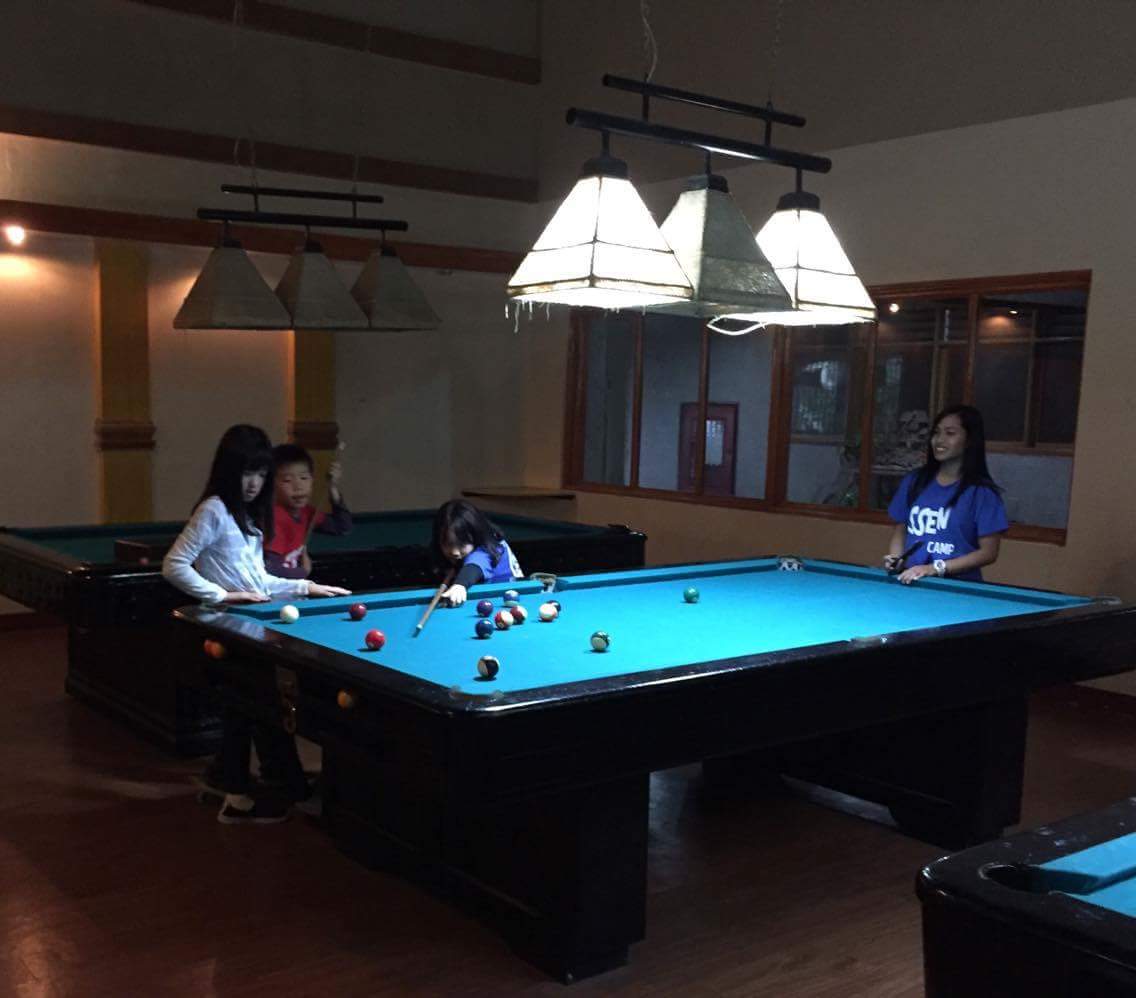In this detailed indoor scene, a group of children and an older lady are gathered around a black pool table with a turquoise blue surface, likely in a game room or a pool hall. The lady, possibly a mother, stands on the right side of the image, identifiable by her long black hair and blue T-shirt with white letters. On the left-hand side of the pool table, three children are visible: a girl with long black hair and a white shirt, a boy with short black hair in a red shirt, and another girl, who is also the one actively playing.

The girl playing pool is leaned over, concentrating as she aims a pool stick towards a red ball, ready to make her shot. The boy in the red shirt and the girl in the white shirt stand close by, watching intently. Above them, a chandelier with three white pendant lights illuminates the scene, casting a focused light on the pool table below. The table itself is scattered with several solid and striped pool balls. In the background, there is a large window providing a view into another room, adding a sense of depth to the setting.